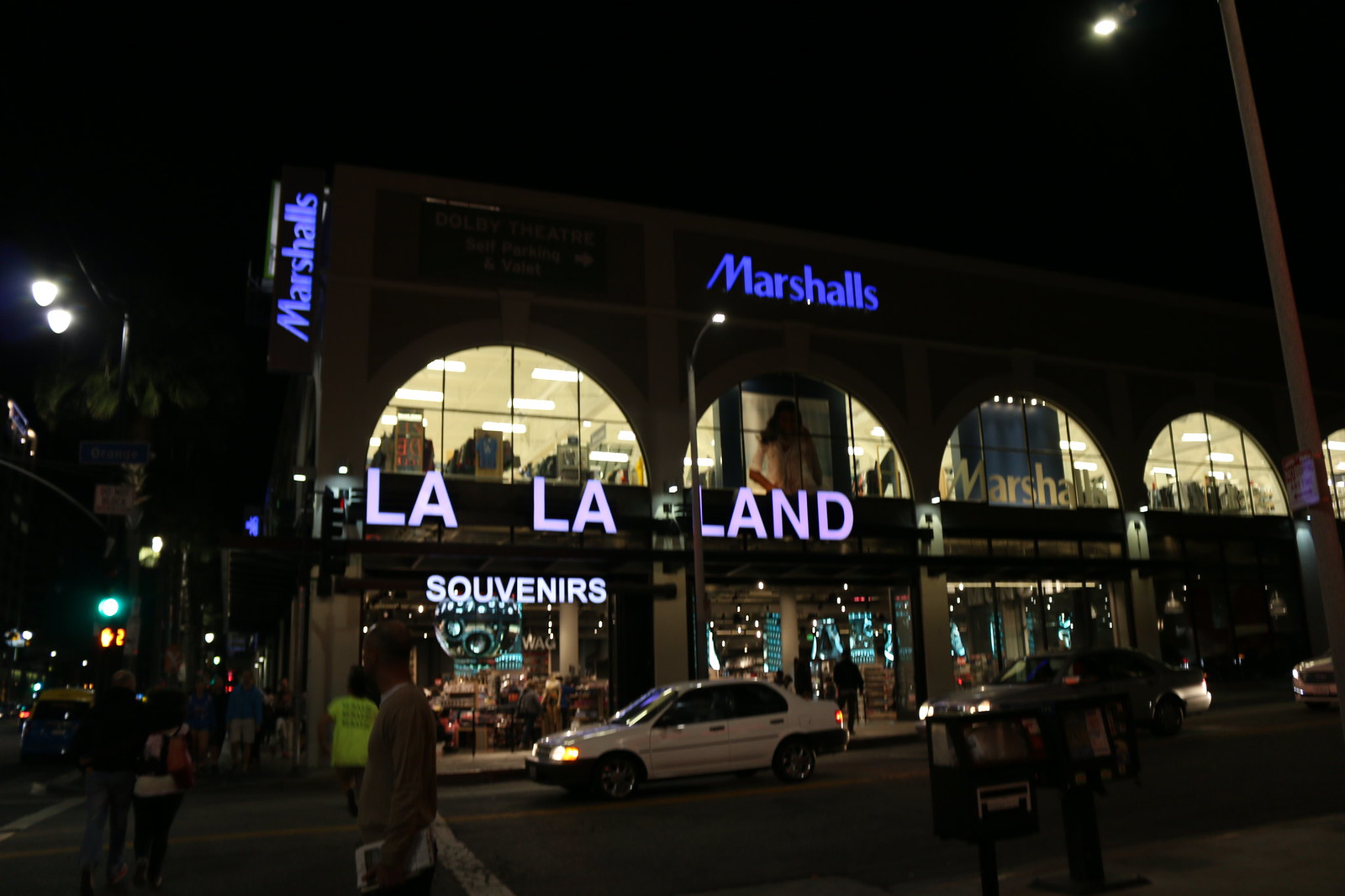The image captures a bustling city street at night featuring a prominent Marshalls store situated at the corner. In the bottom left corner, a crosswalk is visible with various pedestrians; a couple walks away from the viewer, while others stand at the opposite side of the street. The green traffic signal and corresponding countdown timer illuminate the scene, indicating walk time remaining. To the left, partially visible streetlights and vehicles add to the urban atmosphere.

Standing dominant in the background, the Marshalls store showcases its name in two instances: in large blue letters across the top of the second floor and vertically along the left side of the building. The building's second-floor windows reveal aisles of garments and other goods. Between the first and second floors, illuminated white letters spell out "La La Land," while the first floor features bright signage for "Souvenirs."

In front of the store, a white car and several others align, awaiting the traffic light. The bottom right of the image reveals a small section of the sidewalk, adorned with two newspaper vending machines. Streetlights and possibly a palm tree are faintly visible, enhancing the night-time cityscape's ambiance.